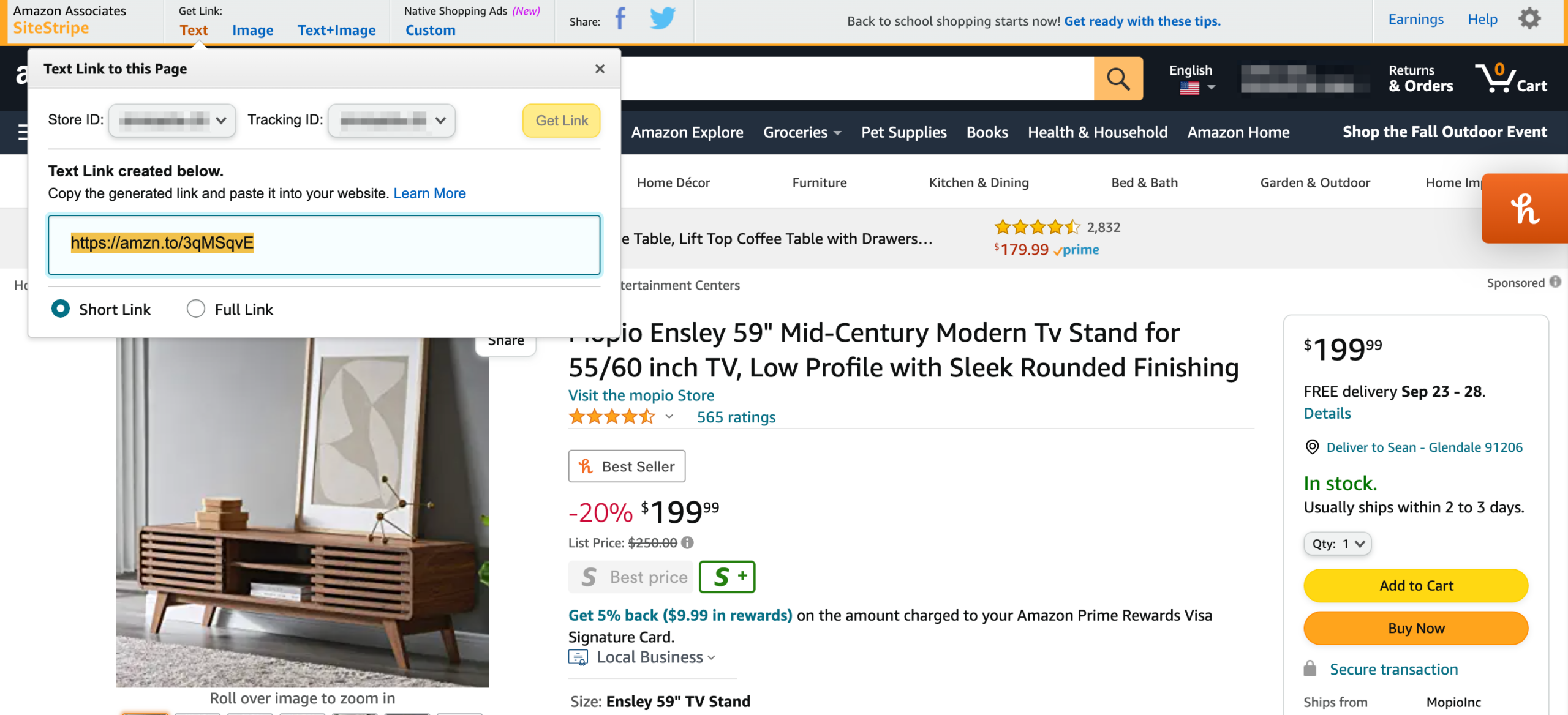The image captures a snapshot of the Amazon website, displaying a product page for a mid-century modern TV stand designed to fit 55 to 60 inch televisions. The TV stand features a low-profile design with sleek, rounded edges and is priced at $199.99. However, it's currently offered at a 20% discount. 

The user has activated a tooltip panel that facilitates creating a short link to the product page. This panel is floating in the top left corner of the screen, slightly obscuring the underlying content. Nonetheless, the TV stand's stylish design, which has a somewhat futuristic appearance and holds various decorative items on its surface, is still visible. At the time the screenshot was taken, the user's cart contains zero items, indicating they have not yet added the TV stand to their cart, implying they are still considering the purchase.